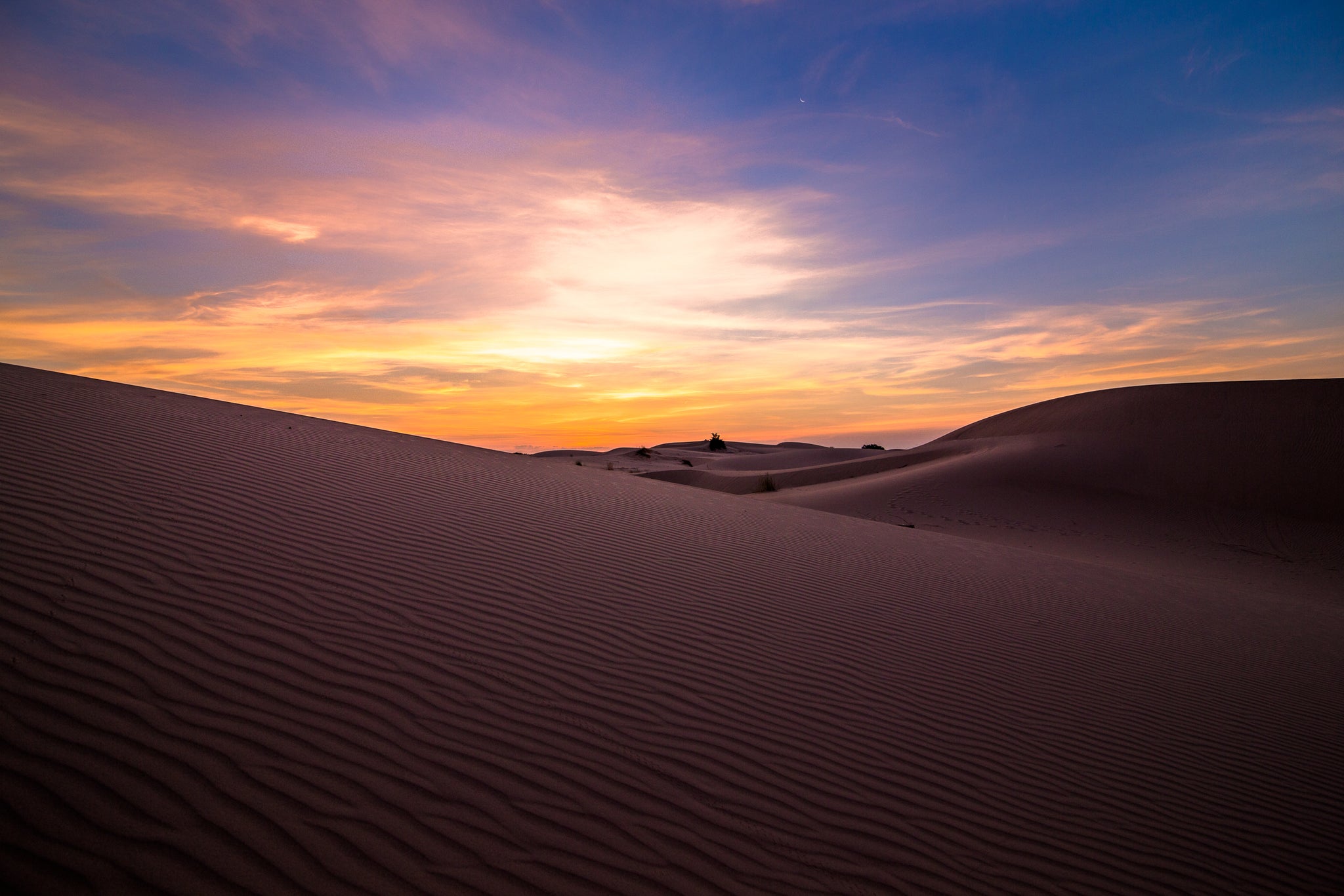The highly professional panoramic landscape photograph captures a breathtaking dusk scene over the hilly expanse of what appears to be the Sahara Desert. Dominating the foreground is a large, rippled sand dune that slopes from mid-left to a third lower right, standing in striking contrast against the dark blues and purples of the surrounding sands. Another gently sloping region rises toward the right, with a valley nestled in between. Distant dunes ripple across the horizon where vibrant orange and yellow hues of the setting sun are adorned with dense, overcast clouds that transition from dark blues and grays at the top to subtly reflecting the sunset's colors below. Amidst these dunes, there are indistinct dark objects, possibly trees or bushes, adding texture and depth to the landscape. The mysterious, stormy atmosphere of the photograph is accentuated by the sun peeking through the cloud cover, casting its final golden light across the tranquil yet dramatic desert scene.